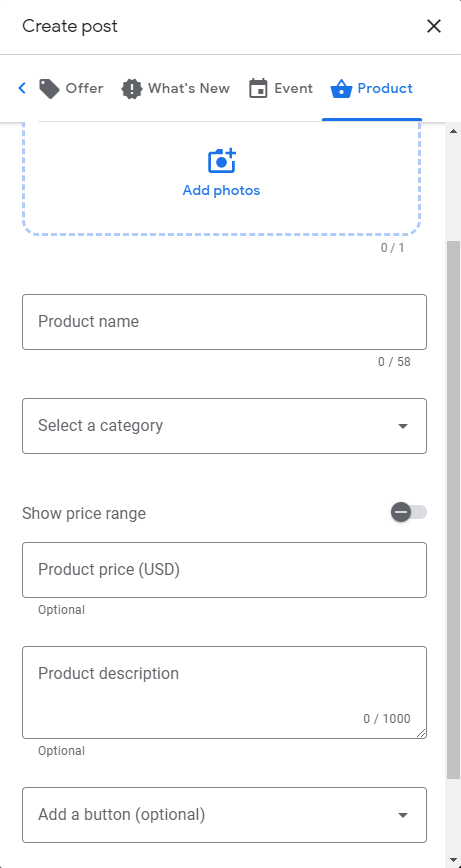At the very top left corner, there is an underlined text saying "Create Post," with an “X” icon located on the far right side of this section. Below, there are several icons and labels:  
1. An image of a shopping tag next to the word "Offer."  
2. A gray circle containing an exclamation mark, followed by the text "What's New."  
3. An image of a calendar alongside the word "Event."  
4. To the right, an icon of a blue shopping cart next to the word "Product."

Beneath these, there is a distinct square outlined with dashed lines labeled "Add Photos." Inside this square is a blue camera icon with a plus sign. To the right of this, in the corner, is the text "0-1."

Below this, there is a large text box labeled "Product Name." Next, there is a drop-down menu labeled "Select a Category," followed by another labeled "Show Price Range." 

Subsequently, a rectangular box is marked "Product Price (USD)." Underneath, there is a note indicating this is optional. 

Another text box is provided for "Product Description," with another optional note underneath it. Finally, there is a rectangle labeled "Add a Button," also marked as optional.